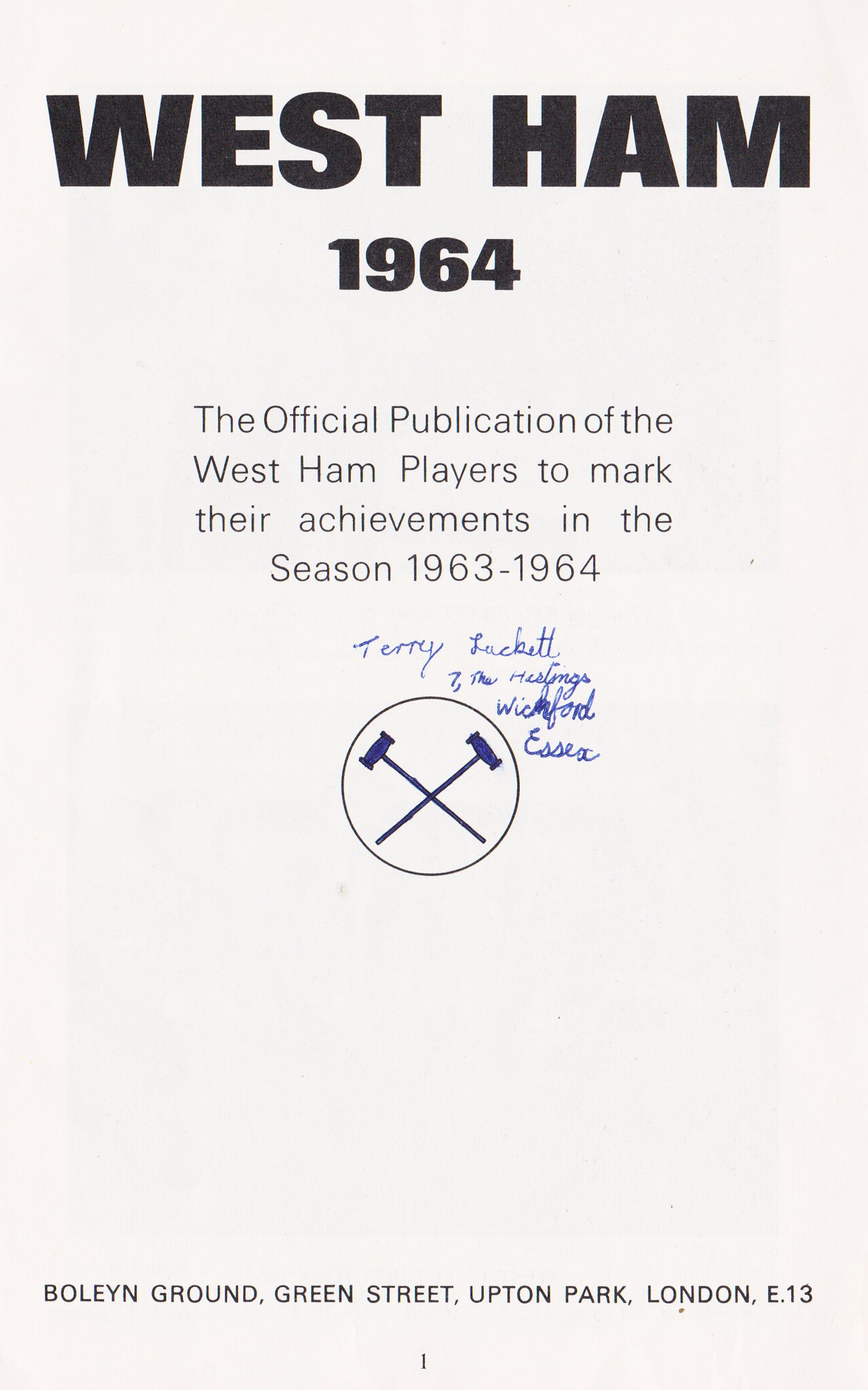The image is likely the cover of a book or a magazine dedicated to West Ham, featuring a simple and clean design on a white background. At the top, in large blocky and bold black font, it prominently reads "West Ham". Beneath that, in slightly smaller bold black font, it states "1964". Following this is a paragraph in smaller text that says, "The official publication of the West Ham players to mark their achievements in the season 1963-1964." Just below this text, there's a handwritten note in blue ink, which seems to read "Terry Luckett, 7, the Hesslings, perhaps Wickford Essex." Central to the design is a circular emblem with two crossed hammers, symbolizing the West Ham team. At the bottom of the cover, there is an additional line of text about the publication's source: "Bowling Ground, Green Street, Upton Park, London, E13."